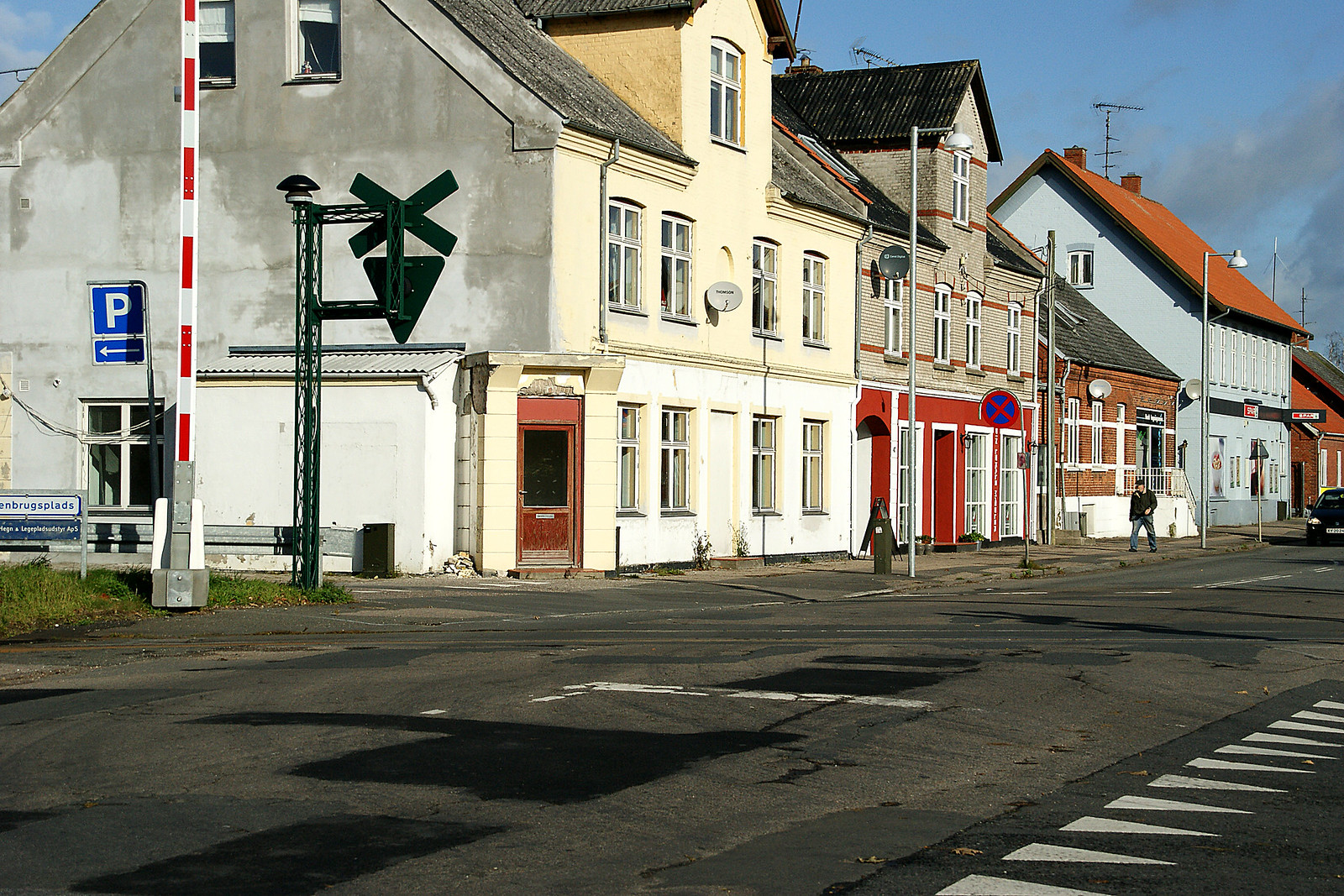This photograph captures a detailed street scene featuring a railroad crossing positioned near a series of diverse buildings. The main perspective is from the road, which is black with white lines and exhibits noticeable wear with cracks and chips. A car can be seen in the distance, and a solitary person is walking toward the camera on the adjacent sidewalk.

The railroad crossing, with its red and white striped gates lifted, cuts across the road prominently, marked by standard railroad signs and signaling devices. A "P" parking sign with a left arrow stands out among the signs on the roadside.

To the left of the road, a row of buildings stands in succession. The closest building, a three-story white concrete structure with multiple windows and a red door, appears aged. Attached to it is a building with a mix of red and tan bricks, followed by a single-story brown brick building with a black roof. Further along, there is a bluish two-story building with a steep red roof.

The sky above is mostly blue, adorned with gray feathery clouds, indicating a clear day. The overall composition highlights the blend of architectural styles and the active yet serene moment of the day.